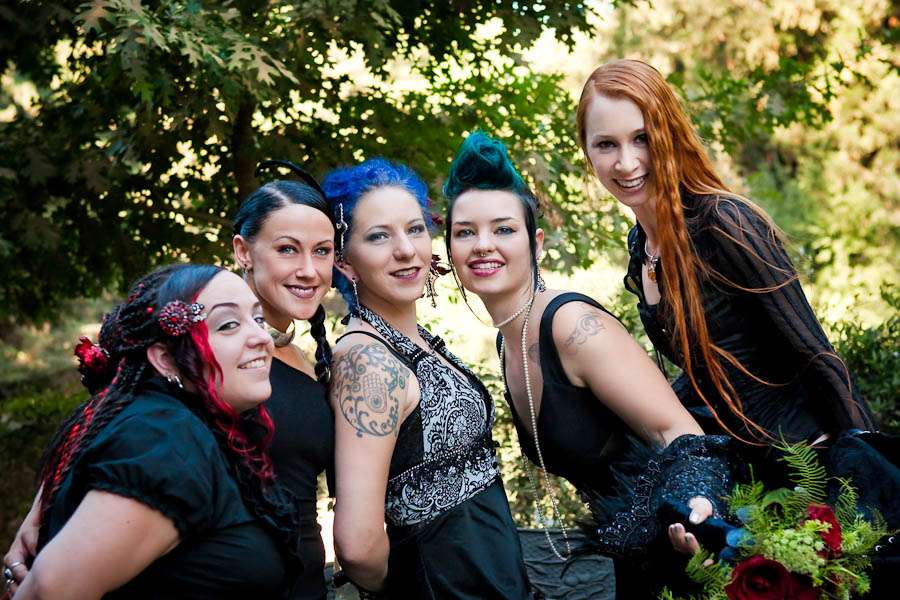In an outdoor daytime setting with a lush, green, tree-lined background, a photograph captures five women posing closely together and facing the camera. Each woman exudes a gothic or emo aesthetic, dressed entirely in black dresses adorned with various jewelry, rings, and tattoos. They all have strikingly pale skin, and their diverse hairstyles add vibrant colors against their dark attire. 

The woman on the far left has long black hair with red streaks. Next to her stands a woman with dark hair styled in a braid. The central figure, possibly the bride given her distinctive blue hair, wears a halter top dress with intricate black and white patterns and proudly displays a tattoo on her upper shoulder. To her right, a woman with a turquoise mohawk holds a bouquet of flowers in her left hand, enhancing the impression that this might be a wedding or special event. Finally, the woman on the far right showcases long, flowing red hair.

All five women seem to radiate happiness, their unique fashion and hairstyles harmoniously blending with their shared gothic style amidst the natural foliage and sunlight filtering through the trees.